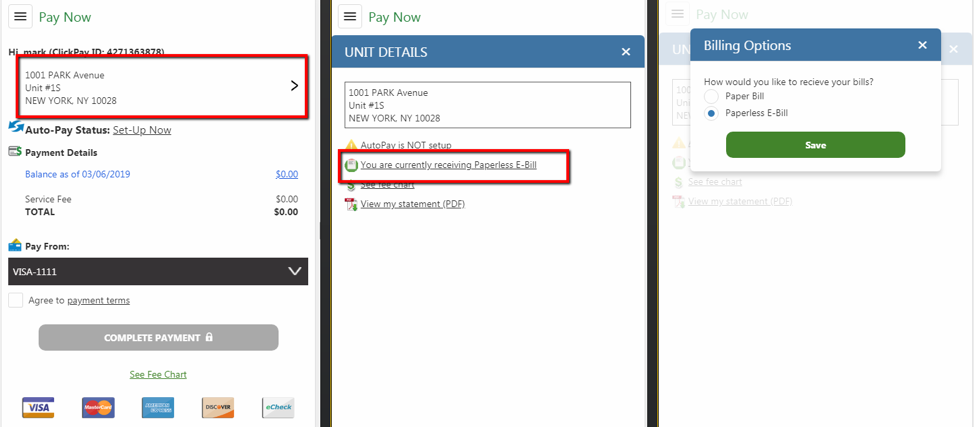This image is a composite of three screenshots related to billing and payment systems, each showcasing different features and options.

The first screenshot displays a payment interface with the following details:
- Payment options include "PayNow," "Highmark," and "ClickPay".
- User ID is listed as "427-136-3878".
- Address: "1001 Park Avenue, Unit 1S, New York, ZIP Code 10028".
- Autopay status is currently set up.
- Balance as of March 6th, 2019, is $0.
- Service fee is also $0.
- Payment is set to be made from a Visa card ending in 1111.
- The "Agree to payment terms" checkbox is not checked.
- The "Complete Payment" button is greyed out.
- There is a notice to "see fee chart" and multiple accepted card types (Visa, MasterCard, American Express, Discover, eCheck) are shown.

The second screenshot confirms that the user is currently receiving a paperless eBill, but Autopay is not set up.

The third screenshot provides billing options, asking the user how they would like to receive their bills:
- First option: Paper bill.
- Second option: Paperless eBill.
- There is also a "Save" button to confirm the choice.

The colors used throughout the images include blue, white, black, grey, yellow, and green.